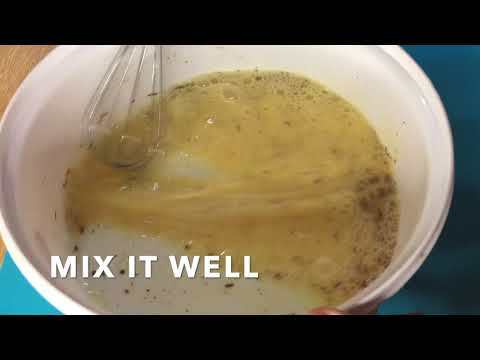This image is a screenshot from a video likely centered around cooking or baking. The photograph features a white mixing bowl, half-full with a yellow and white liquid mixture, perhaps resembling eggs combined with milk and possibly some powder or cinnamon. A small metal whisk rests inside the bowl, leaning against its side, actively involved in mixing the contents. The bowl is set on a blue cloth, presumably to prevent spillage, with traces of a brown wooden surface peeking out from the upper left corner. The image has a letterboxed appearance with black bars at the top and bottom, along with the text "MIX IT WELL" prominently displayed in white, capitalized letters in the lower left corner. The overall scene suggests someone in the midst of preparing a food dish, potentially pancake batter or a similar concoction.